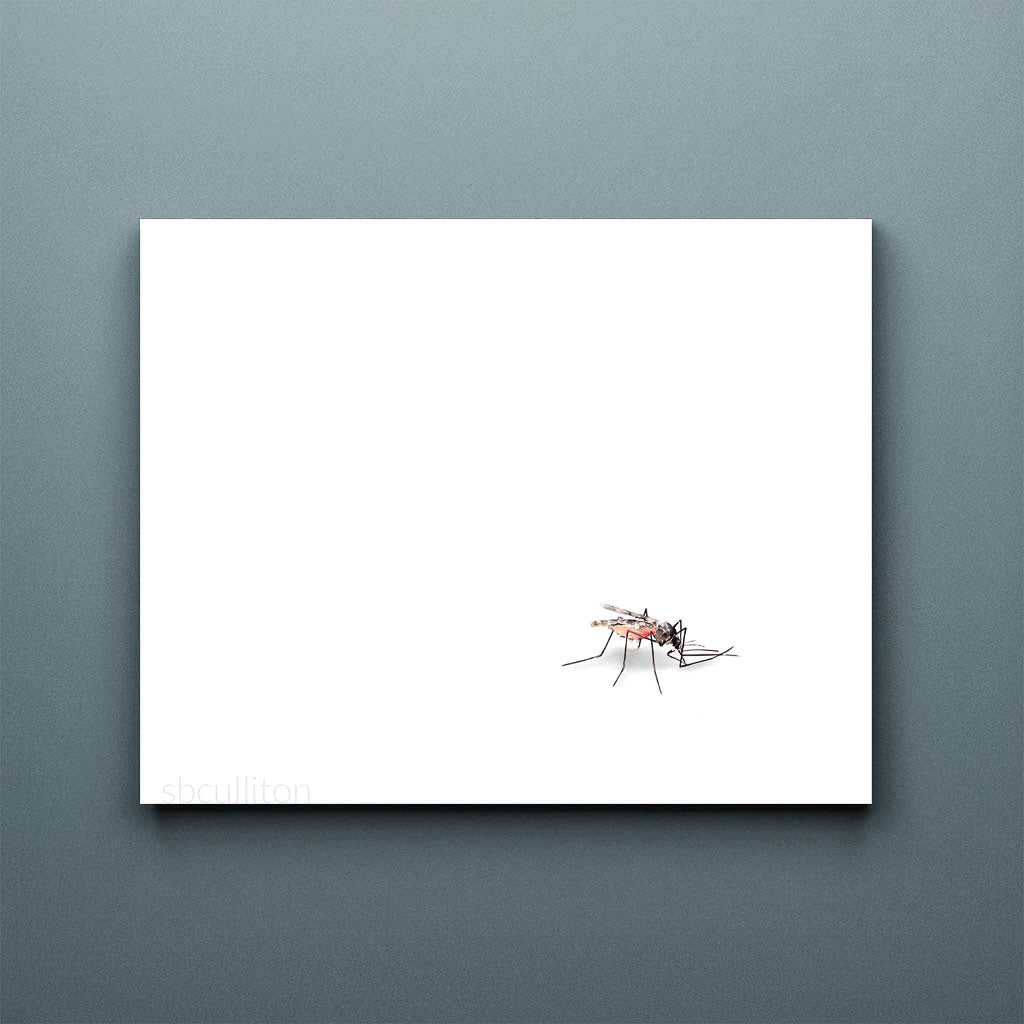The image depicts a minimalist artwork prominently positioned against a gray backdrop, presenting a contrast between its light and dark shades. The backdrop is gray with a slightly darker bottom half, and the central focus is a rectangular white box, perfectly centered both vertically and horizontally. Within the lower right quadrant of this white space resides the detailed illustration of a mosquito. The mosquito features long black legs and a distinct black stinger. Its underbelly showcases a light pink hue transitioning to a darker pink or red near its head, indicating it may have fed recently. The wings are delicate and appear gray and translucent, adding to the intricate depiction. The overall composition, with no additional text or elements, emphasizes the simplicity and detail of the insect, which seems poised or caught in a moment, ready to be swatted.